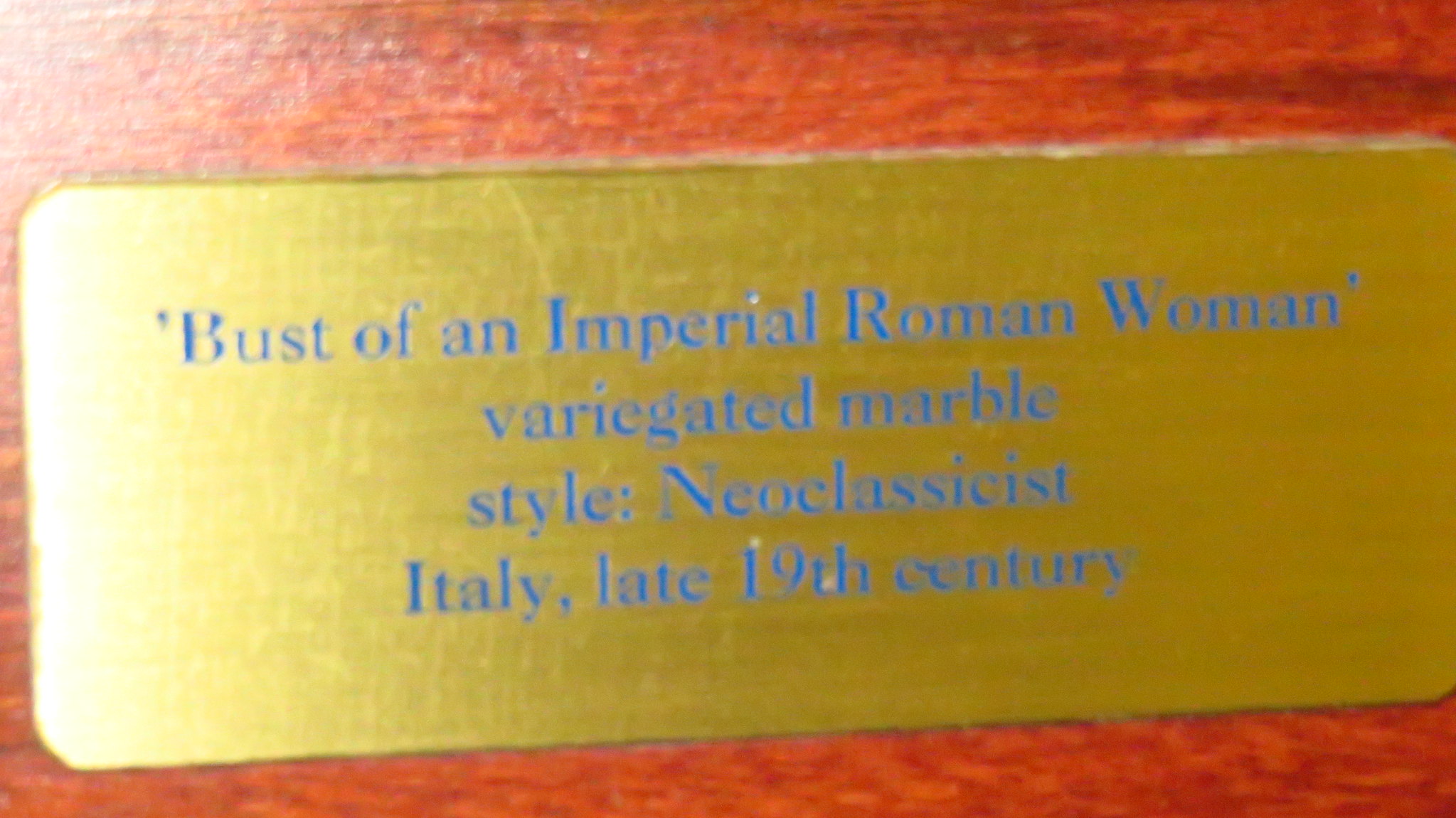The image is a detailed close-up of an aged, gold-colored plaque with scuffs and signs of wear, set against a reddish wood background with visible wood grain. The plaque, reflecting a distinct light source primarily in the top left corner, is inscribed with blue text that reads: "Bust of an Imperial Roman Woman, Variegated Marble Style, Neoclassical Italy, Late 19th Century." The setting appears to be an old-fashioned environment, likely a museum or similar institution, indicating an English-speaking country due to the language of the inscription.